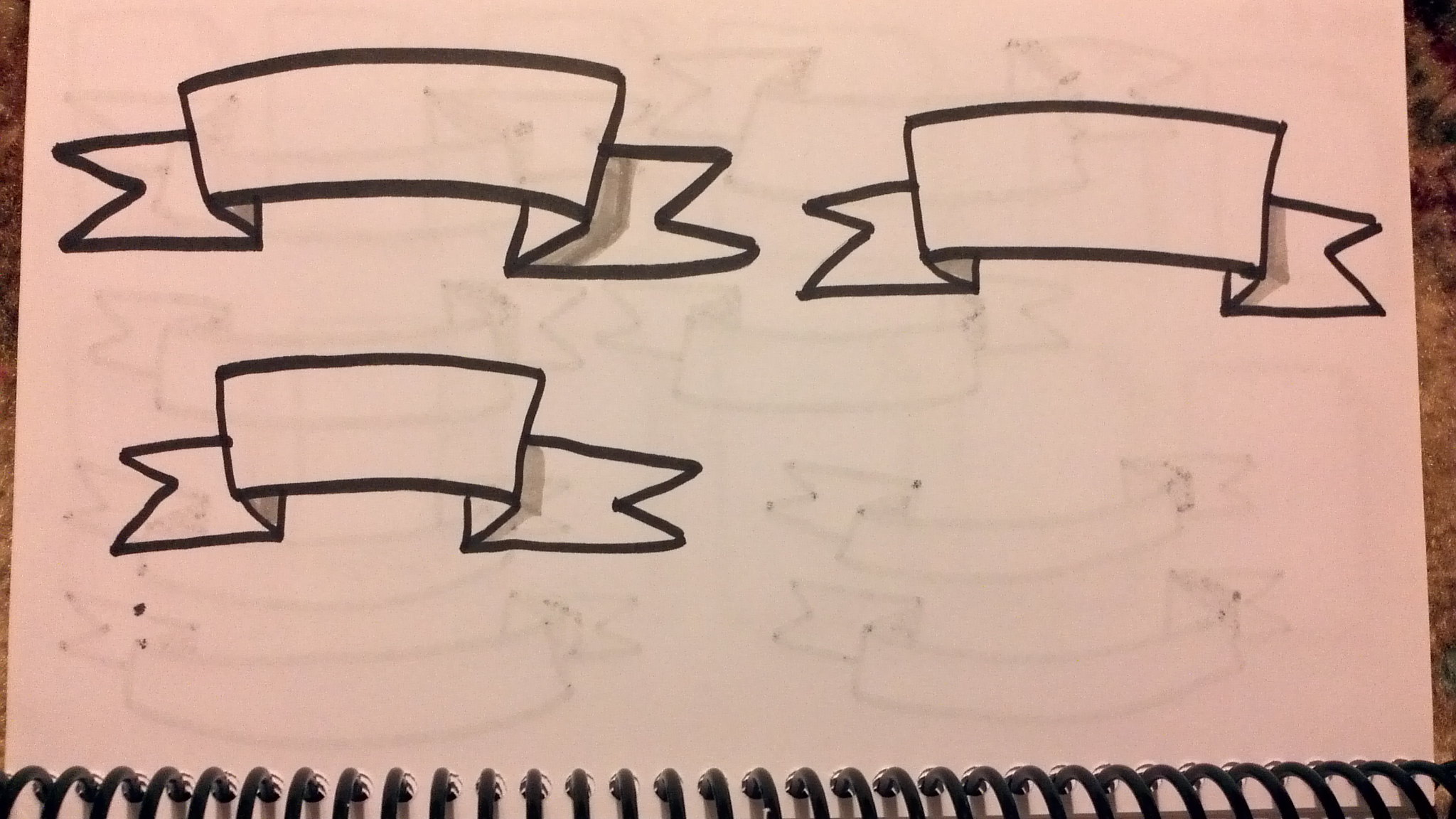The image showcases a piece of solid white paper attached to a black ring binder, positioned so that the binder rings are at the bottom and the paper rests on top. On the paper, there are several hand-drawn illustrations resembling 3D labels. Each label has flattened sides, with the center portion raised into a rectangular shape, reminiscent of a nameplate. There are three such labels on the page: two placed side by side near the top, and a third one situated below the first label. While they are generally of similar size, the first label is the largest.

The paper is somewhat transparent, revealing faint, partial outlines of additional 3D labels on the verso. It appears that there are numerous similar drawings on the reverse side, with an estimated six or seven visible through the paper.

The notebook is set against a partially visible table with a unique brown and black marbled pattern, glimpsed along the right and left edges of the image. This setting provides a contextual background for the sketched notebook.